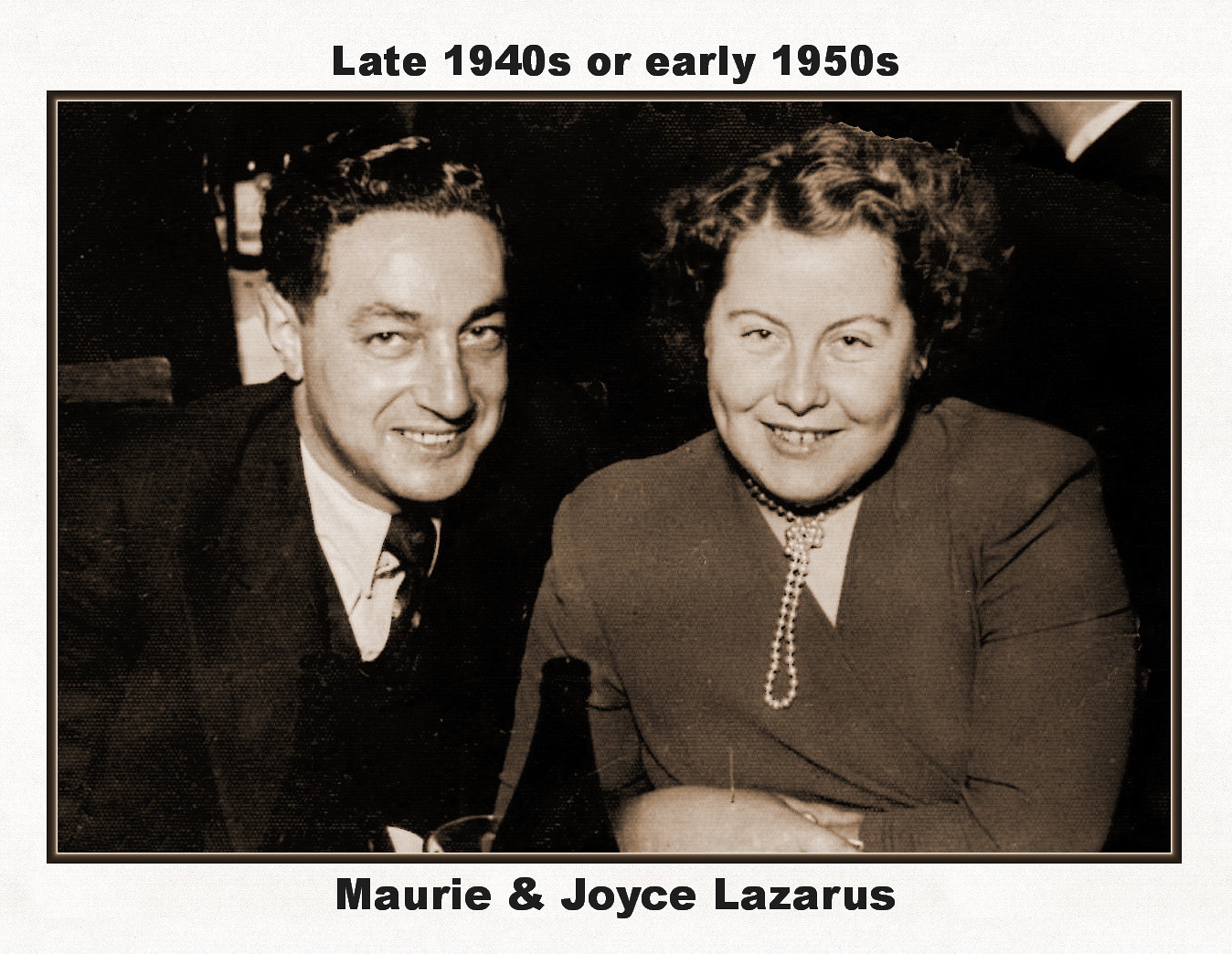The image is a vintage black-and-white photograph, framed with a black border. The central feature of the image is a couple, identified as Maury and Joyce Lazarus, positioned directly in the center. The man, Maury, is on the left, smiling, with black hair and dressed in a gray or black suit, white shirt, and a gray and black tie. The woman, Joyce, is on the right, also smiling, with short, curly brown hair, wearing a pearl necklace and a gray dress. The couple appears to be indoors, with a mostly black background. There is a glass bottle placed between them. Additionally, in the background behind the man, another figure is visible, dressed in a black suit and white shirt. Text outside the image border at the top reads "late 1940s or early 1950s," and at the bottom, it identifies the subjects as "Maury and Joyce Lazarus." The entire scene is captured in shades of black, white, and gray.